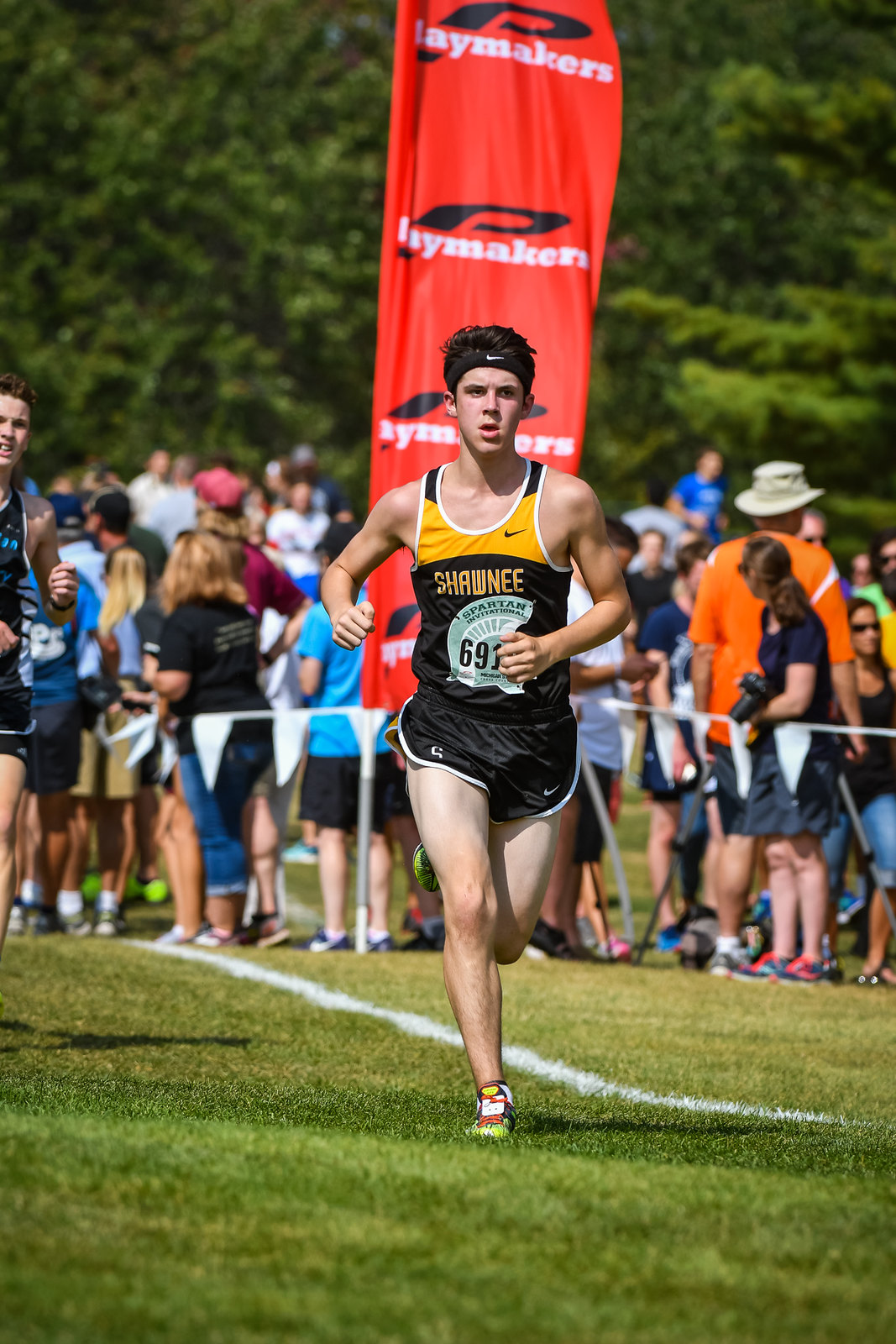In this vibrant image of a marathon race event, we see a focused runner in the foreground. He is a young white male with short brown hair, wearing a headband and a black sleeveless jersey with yellow accents at the top and white outlines, emblazoned with "Shawnee Spartan Invitational 691" and the Nike logo. He is also wearing black shorts. His serious expression highlights the intensity of his run across a green grassy field, marked with a white line. 

Partially visible behind him is another runner, also in a sleeveless jersey, though the details are less clear. This second runner is further back and slightly cut off from the frame. Surrounding the runners is a large crowd of spectators, cordoned off by a rope with various small flags. The spectators, dressed in summer attire such as shorts and hats, are intently watching the competitors, though some are looking in different directions.

Dominating the background are tall green trees, their leaves filling the scene with lush color, suggesting a bright, sunny day. Prominently, there is also a large red banner behind the main runner, with partially visible writing that likely reads "Laymakers." The overall ambiance of the image depicts a warm, bustling, and spirited race day.